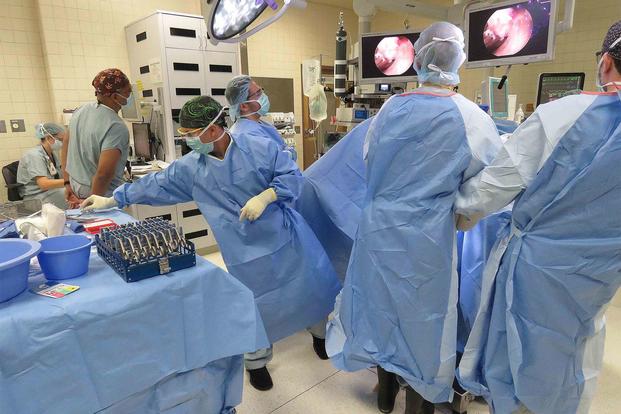This detailed photograph captures an active operating room, meticulously arranged for surgery. On the left side of the image, there is a table draped with a blue cloth, hosting an assortment of surgical tools, including blue buckets, a blue rack with silver instruments, and a flat red object. The table is accompanied by various medical supplies, such as IV bags, a gas or oxygen tank, and a bright overhead light illuminating the scene. 

To the right of the table, a team of six medical professionals is intensely focused on an operation. All members of the team are clad in blue surgical gowns, masks, and varying types of headgear. Four appear to be doctors, distinguished by their positions around an operating table, although the patient is obstructed from view. Two additional figures, likely nurses, wear a lighter shade of blue. One of these nurses is seated at a desk with a computer, while the other stands beside her. 

Above the medical team, two black monitors display detailed, zoomed-in images of the inside of a patient’s body, aiding the surgical process. The scene is highly organized, with surgical precision evident in the arrangement of the tools and the team's focused demeanor. The operating room’s background features white tile flooring, beige-tiled walls, and large cabinets, adding to the sterile and controlled environment essential for surgical procedures.